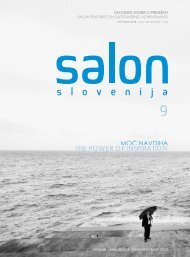This magazine cover features a striking grayscale image with a white, cloudy sky blending into a dark, expansive ocean at the bottom. A small figure of a person, dressed in a suit and holding an umbrella, stands near the bottom edge, possibly on a dock, gazing upwards. The title “Salon Slovenija” is prominently displayed at the top in large blue text, with a smaller number "nine" positioned to its bottom right. Above the title is some small gray text. In the middle of the cover, over the ocean, is another blue text that reads “The Power of Inspiration.”